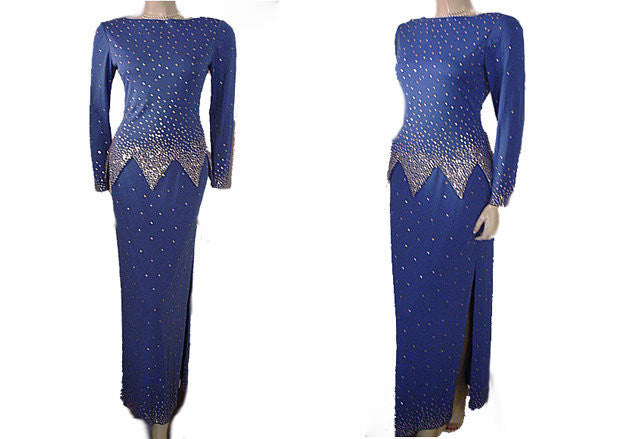The image showcases two photographs of the same blue dress, presented against a white background. The dress, adorned with shimmering glitter or polka dots, is displayed on a featureless mannequin body that lacks a neck, legs, and, in one view, hands. The garment features long sleeves and has a prominent design element where the dots increase in density from the top down to the waist, creating an almost white appearance in the middle section. The top part of the dress resembles a tunic, ending in a distinctive triangular fringe. In the left photograph, the mannequin is positioned facing directly forward, allowing a clear view of the dress's front, which includes a horizontally cut neckline. The right photograph provides a three-quarter view from the back right, highlighting a high slit on the side that extends nearly to the hip. Both images emphasize the dress's intricate detailing with gems spread throughout, creating a brilliant, eye-catching effect.